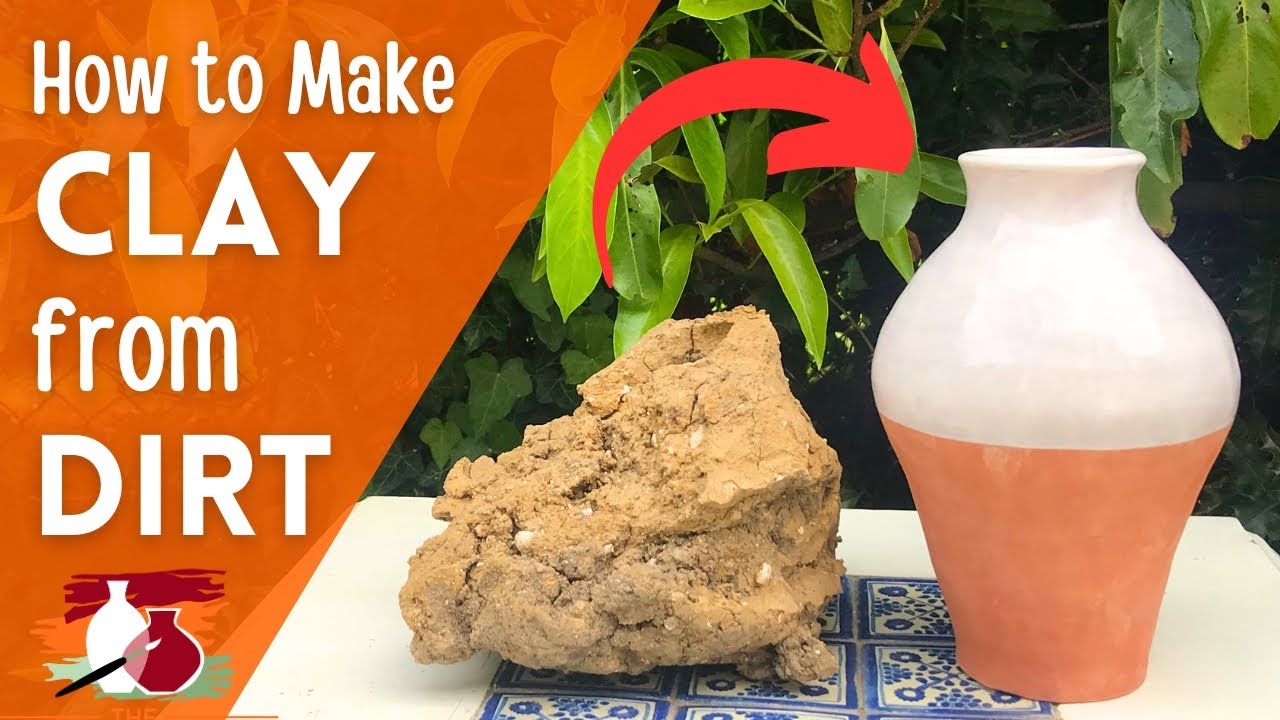The image features an instructional advertisement with an orange trapezoidal banner on the left side that reads "How to Make Clay from Dirt" in white font. Below the text, there is an illustrated image showing two clay pots, one being painted red with a paintbrush. Moving to the right side of the image, there is a real-life example of a chunk of clay, brown with white specks, placed on a white table that has a blue floral tile pattern in the center. A red arrow points from the clay to a beautifully finished vase, which is peachy pink on the bottom and white on the top. In the background, lush green tree leaves hang, indicating that the image was taken outdoors.